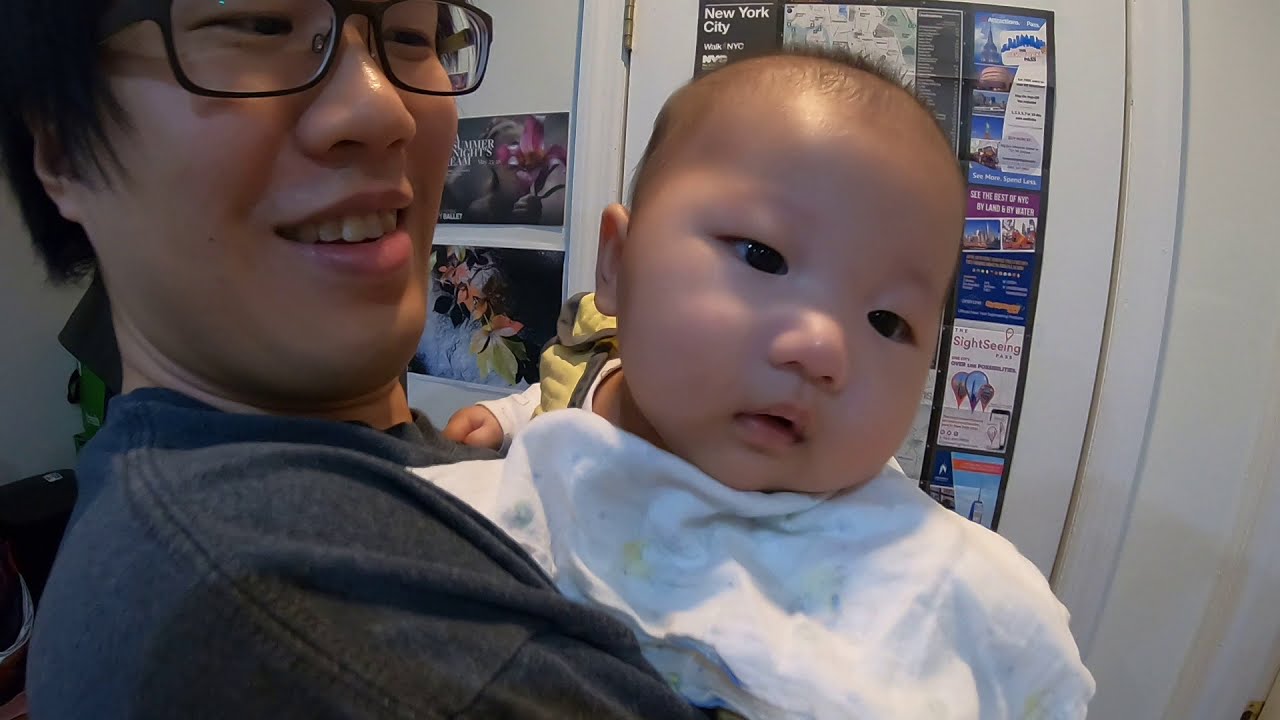A tender photograph captures an Asian baby, estimated to be around six to eight months old, nestled in the arms of a person who appears to be the baby's father. The father, a middle-aged man with black glasses, is smiling as he looks lovingly at his child. He is dressed in a grayish-blue shirt and stands to the left of the baby, who is wrapped in a soft, white blanket. The baby, with thin, short hair and wearing a white shirt, gazes off to the right with its head slightly tilted. A yellow bib with a brown border is snapped over the baby's shoulder, partially visible beneath the blanket. In the background, the scene is set against a door and a white wall adorned with multiple posters. One poster prominently displays "New York City," while other posters, though illegible, add colorful floral imagery to the setting. The overall warm atmosphere suggests an indoor environment filled with love and visual interest.